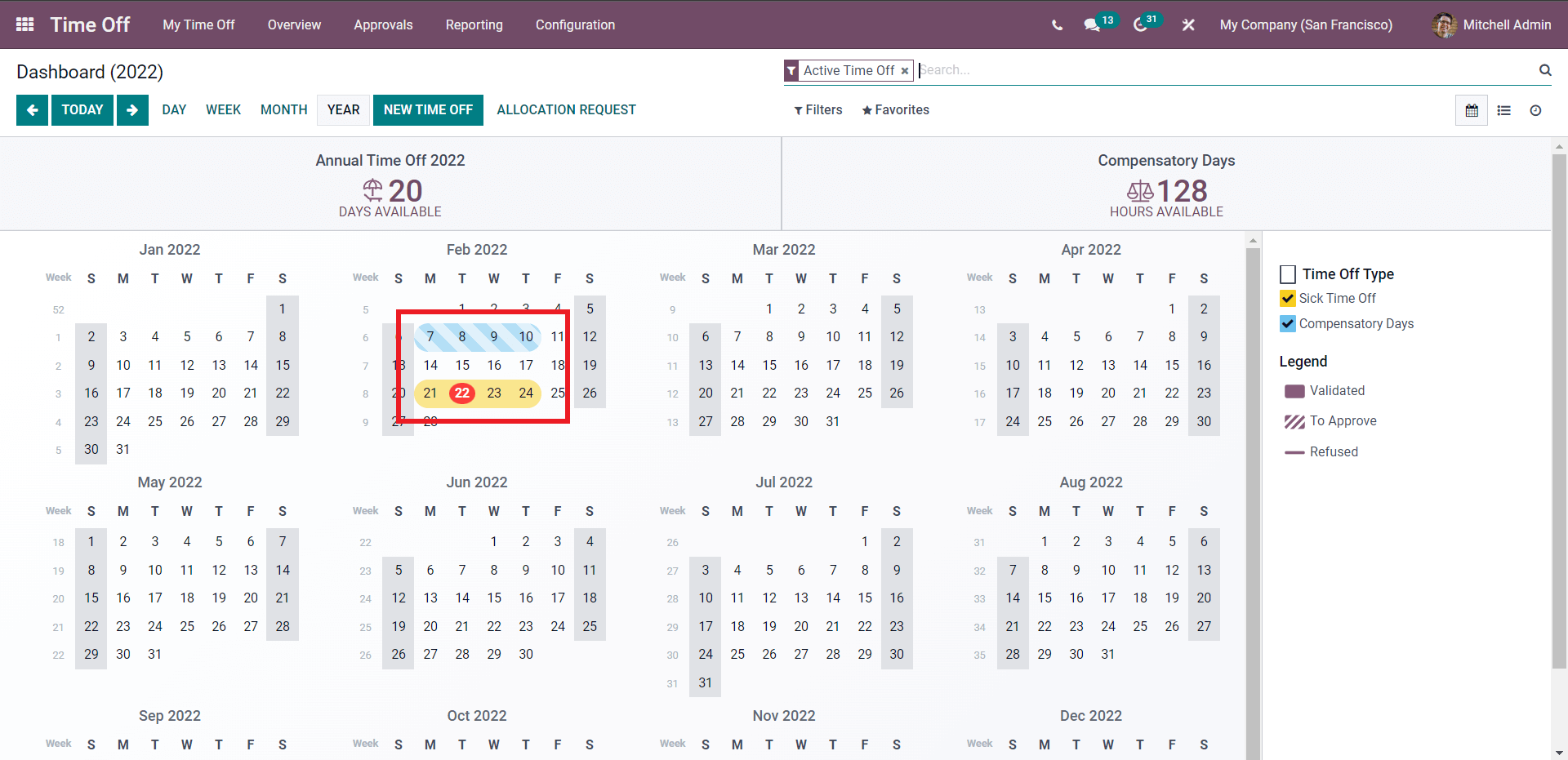This screenshot features a detailed, user interface from a time-management application. At the top, there is a dark plum header with white text presenting the navigation options: "Time Off," "My Time Off," "Overview," "Approvals," "Reporting," and "Configuration." On the far right of the header, a message icon displays the number 13 in a green oval, followed by the text "My Company San Francisco." In the upper right corner, there's a profile picture of a man with glasses and dark hair labeled "Mitchell Admin."

Below the header, on the left side, there is a section titled "Dashboard 2022." Beneath this is a green box labeled "Today," flanked by left and right arrows for navigation. Adjacent to this, the options "Day," "Week," "Month," and "Year" are presented in black text on a white background. To the right, there is another green box labeled "New Time Off."